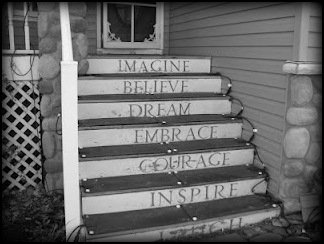This black and white photograph features a wooden house with stone or rock trim, showcasing a staircase leading up to a front porch. The porch includes a white banister and a front door fitted with a screen door adorned with floral decor in its lower corners. The wooden steps are each painted with encouraging words on a white background in light black text. From top to bottom, the words read: Imagine, Believe, Dream, Embrace, Courage, and Inspire. The final step is weathered and unreadable. The scene also hints at a window positioned above the steps, contributing to the homey feel of the entryway.